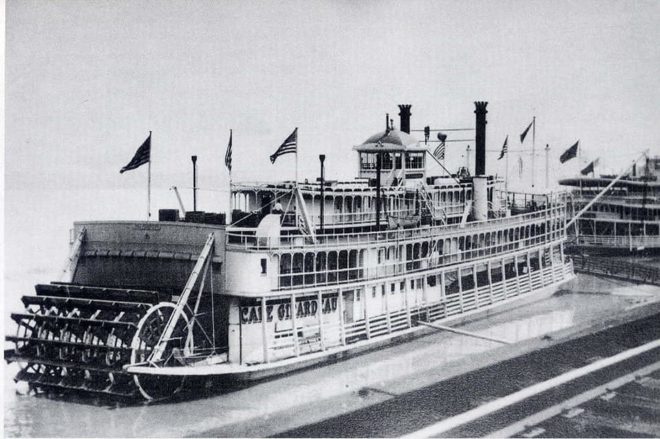A historic black and white photograph, estimated to be over 100 years old, captures a large, classic-styled paddle boat named "Cape Girardeau" docked with a long wooden plank extending from the dock across a thin line of water to its lower deck. The riverboat, which appears white in color, displays three levels including a base, a middle deck, and an upper deck with a small pilothouse, likely used for navigation. At the rear of the vessel, the paddle wheel is visible, hinting at its propulsion method. The boat is adorned with numerous flags, including at least three American flags prominently displayed at its corners and edges. The structure also features two black smokestacks positioned behind the bridge. Despite the clarity of the vessel's features, no passengers are visible aboard. In the blurred background, another riverboat can be seen, adding depth to the historic river scene.